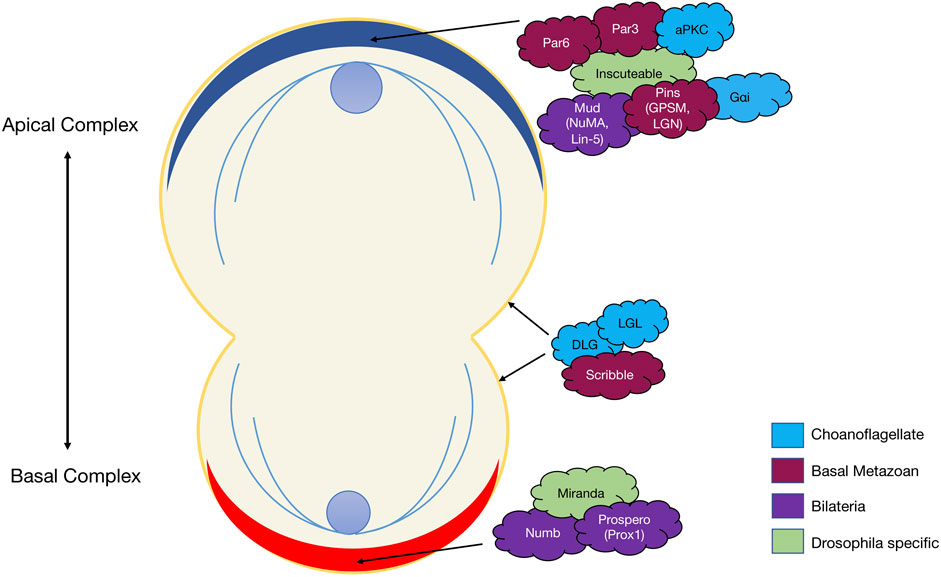The image is a detailed schematic illustrating the structure of the brain, featuring specific terminologies and color codes in the lower right corner. The color codes are as follows: light blue represents choanoflagellate, dark purple indicates basal metazoan, purple signifies bilateria, and light green denotes drosophila-specific elements. Central to the schematic is an inverted figure-eight shape with distinct parts. The upper loop of the figure-eight is larger and colored blue, while the lower loop is smaller and colored red. An arrow on the left side of the image labels the top as the apical complex and the bottom as the basal complex. The schematic also includes various color-coded arrows originating from colored clouds, which point to different sections of the figure-eight, suggesting specific structures within the brain.